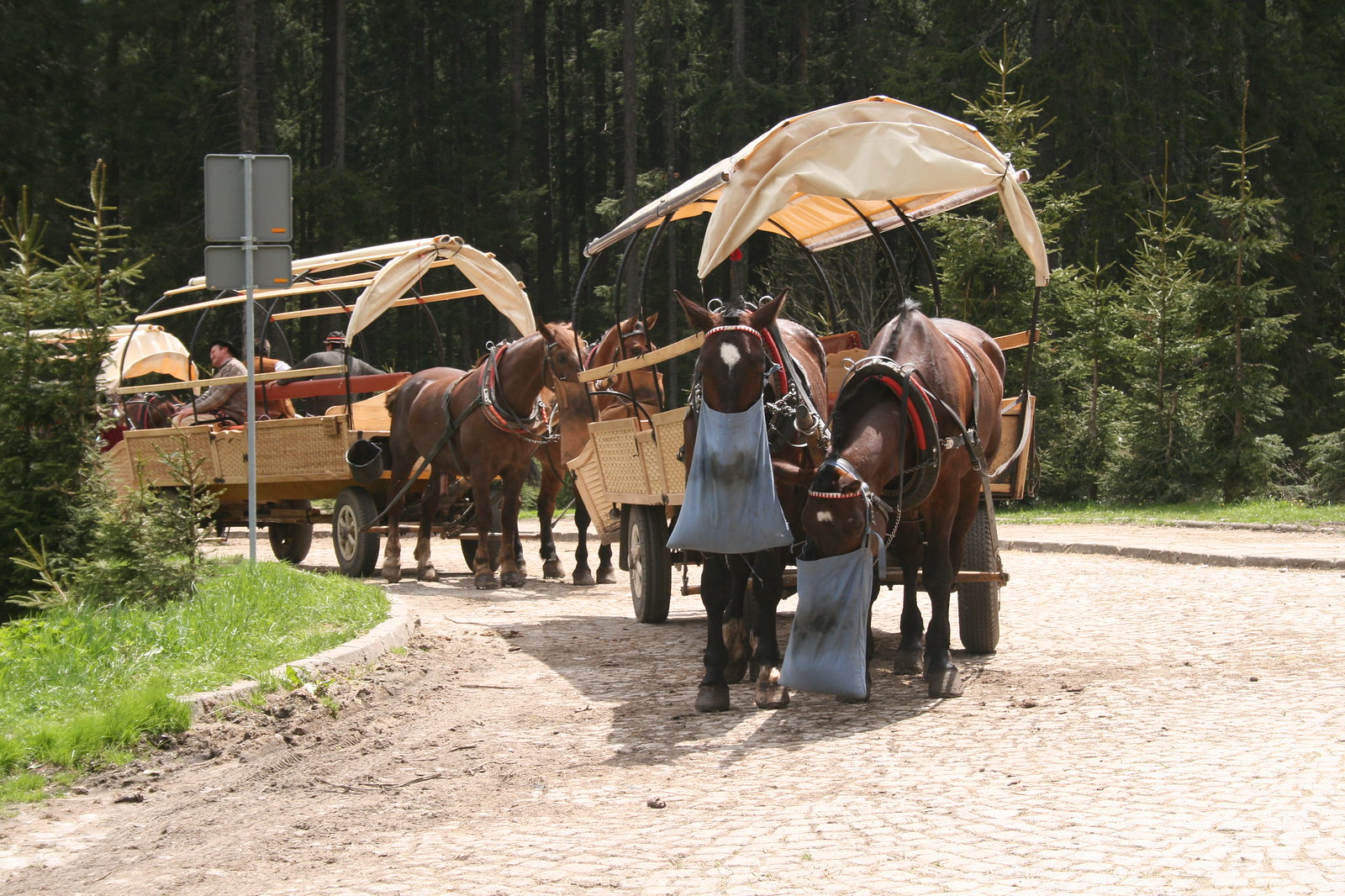The image depicts a picturesque scene of two horse-drawn carriages traveling along a stone road with a grassy verge to the left, accompanied by a road sign facing away from the viewer. Majestic, tall pine trees densely populate the background, indicating a deep wooded area, possibly in a mountainous region. Each carriage is drawn by two brown horses adorned with light blue, slightly dirty feed bags over their faces, taking a break and munching on some oats. The carriage in the front, which appears empty, has a beige top cover and basket-like edges. In contrast, the second carriage seems to be carrying three or four people, resembling the type used for tourist rides with its long, wooden structure and open top. Despite having a vintage appearance reminiscent of the Oregon Trails, the photograph's modern quality shines through. The horses are seen walking towards the camera, their carriages journeying along a dirt road and possibly rounding a corner.